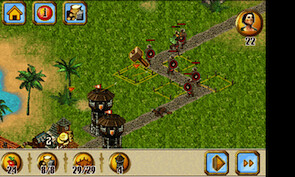This detailed screenshot captures a moment from an engaging computer game. The scene features a gray zigzagging path traversing a meticulously rendered green landscape. Along this path are two defensive towers and a majestic castle, flanked by two tall palm trees. A serene blue body of water adds a touch of tranquility to the vibrant setting.

On the path itself, there are small armored figures carrying shields, suggesting an ongoing battle or quest. Hovering above is a large hammer, seemingly ready to strike at any moment. Above the castle, several gleaming gold coins float in the air, possibly representing in-game currency or rewards.

The top of the screen is adorned with a user interface displaying various icons. Starting from the left, there's a house symbol, a coin symbol, and a third box containing an unrecognizable symbol. In the top-right corner, a round gold coin featuring a man's face is displayed next to the number 22, which likely denotes the player's current coin count.

This descriptive caption should provide a clear and immersive visualization of the game scene for those who have not seen the image.